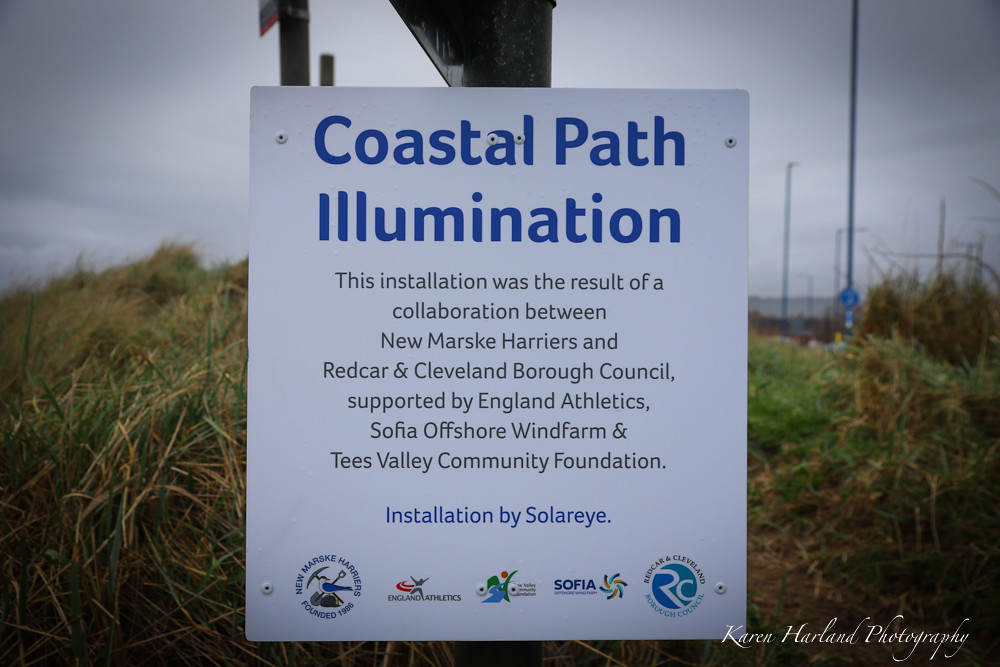The photograph depicts an informational sign installed outdoors in a large grassy field with a mix of green and yellowish hues. The background features a gray, overcast sky with dark clouds and faint outlines of electric poles and possibly trees or street lights. The white square sign is mounted on a black pole and prominently displays "Coastal Path Illumination" in bold blue text at the top. Below, in black text, it states that the installation is the result of a collaboration between New Marsk Harriers and Redcar and Cleveland Borough Council, supported by England Athletics, Sophia Offshore Wind Farm, and Tees Valley Community Foundation. At the bottom, in blue text, it credits the installation to SolarEye, accompanied by sponsor logos for New Marsk Harriers, England Athletics, Sophia, and Redcar and Cleveland. The bottom right corner of the image is marked with the credit "Karen Harland Photography."